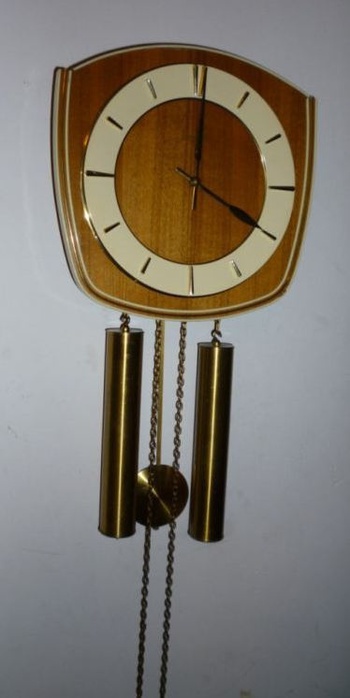This color photograph captures a distinctive wall-mounted pendulum clock with mid-century modern design elements. The clock is rectangular with slightly rounded top corners and rounded bottom corners, giving it a shield-like shape. Its wooden backplate features brass trim around the edges, emphasizing its stylish appearance. The white clock face, also bordered in brass, lacks traditional numbers, instead showcasing sleek brass hour markers: larger dashes at the 12, 3, 6, and 9 positions, and smaller dashes for the remaining hours. Two long black hands indicate the time without the inclusion of a second hand.

Beneath the clock face, the classical design elements become evident. Two brass chains and weights hang symmetrically on either side of a central brass pendulum, hinting at the clock's chiming mechanism. The overall aesthetic combines the clean lines and material contrast typical of mid-century modern design with the functional charm of an old-fashioned chiming clock. The clock is mounted against a white wall, with only a slight gap between its top and the wall edges on either side, highlighting its prominent presence.